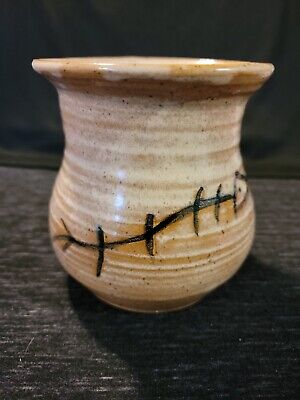This photograph features a small antique pot, approximately 3 to 4 inches tall, with a light brown and beige horizontally striped surface. It rests on a mottled black and white surface, while a blurred black backdrop creates depth to the image. The pot’s shape includes a gently curved bottom, a flat base, and indented sides that smoothly curve out towards the top, finishing with a glossy brown rim. The entire surface of the pot is highly reflective, catching light particularly on the front left side.

Accentuating the pot's surface is a distinctive design that arches from the bottom left to the top right. This design comprises a slim black line forming a shallow S shape, punctuated by four short black dashes. Towards the left end of this line, there's an arrow-shaped mark made up of two lines at a 45-degree angle, pointing right. On the right end, the line concludes with a small black triangle, also pointing to the right.

Additionally, the overall look of the pot suggests it is a very old, possibly antique piece, with a pattern around it that appears to be somewhat circular. The described black markings on the surface somewhat resemble stitches or tally marks, adding a unique and intricate detail to its decoration.